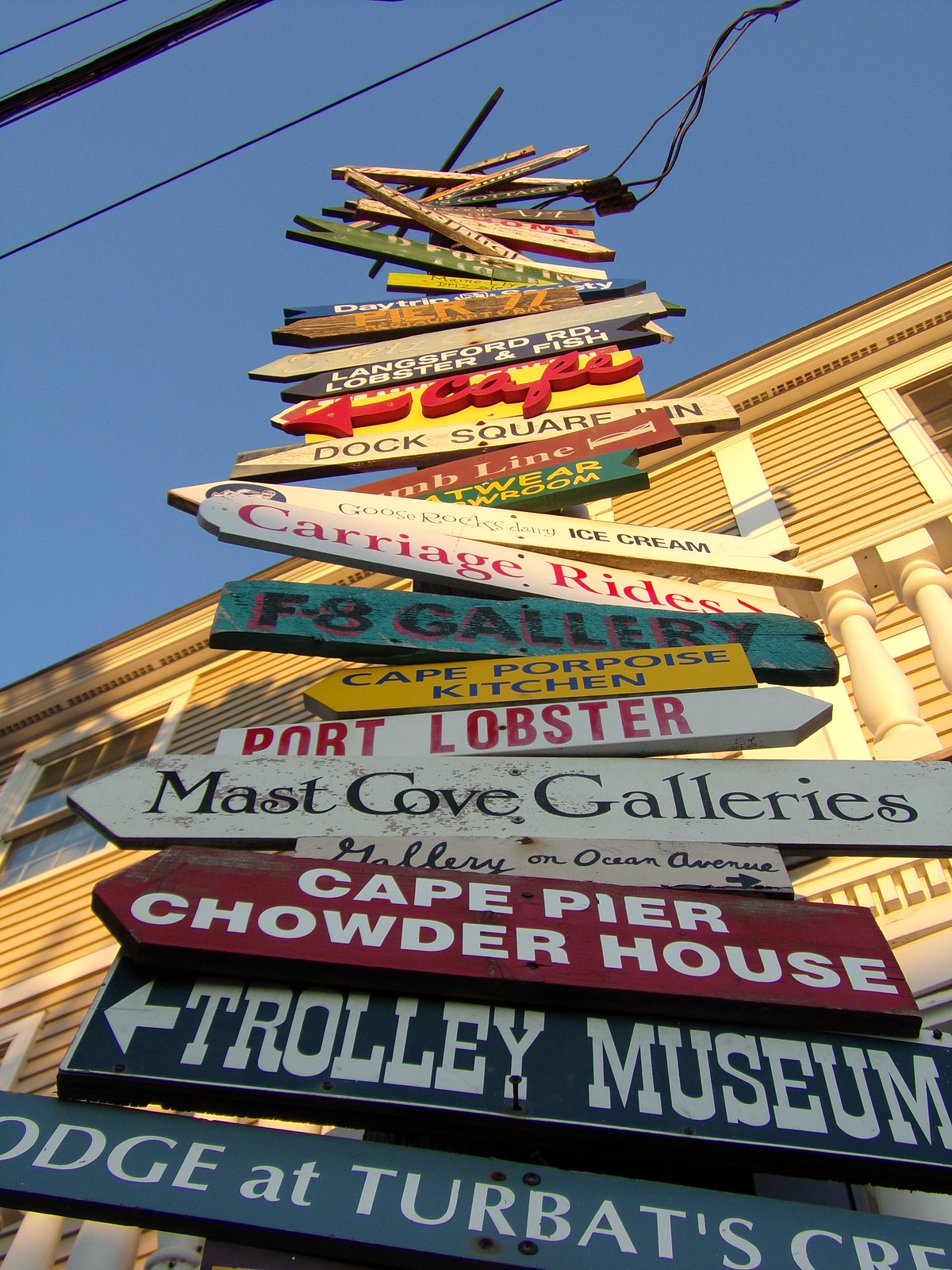This vertically oriented photograph showcases an outdoor scene in front of an ornate yellow wooden building. The image captures a tall stack of around 25 narrow, pointed wooden signs, each pointing in different directions, guiding viewers to various local attractions. From bottom to top, the signs list "Dodge at Turbats" (blue and white), "Trolley Museum," "Cape Pierce Chowder House," "Mast Cove Galleries," "Port Lobster," "Cape Porpoise Kitchen," "F8 Gallery," "Carriage Rides," "Ice Cream," "Lamb Line," "Dock Square Cafe," "Langsford Road," "Lobster and Fish," and "Pier 27 or 77." The signs extend all the way up, silhouetted against a clear blue sky, adding charm to the picturesque street.